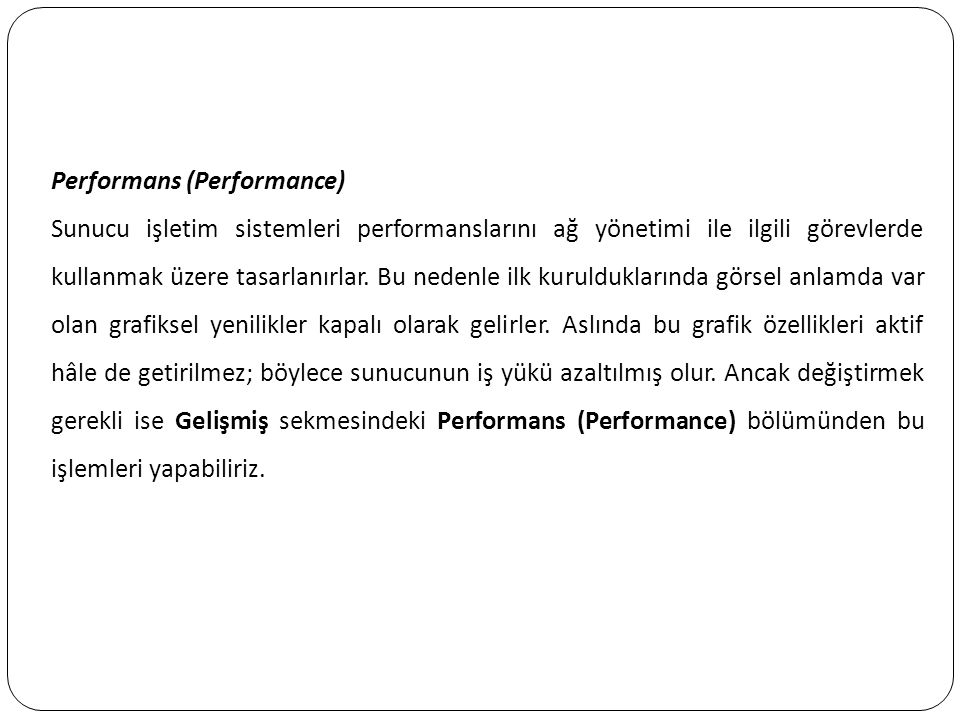The image displays a block of typed text on a white background, surrounded by a thin black rectangle with rounded corners. The text itself is predominantly in a language that appears to be either Middle Eastern or Eastern European, featuring several instances of the English word "performance." The heading at the top is bolded and reads "performance" followed by the same word in parentheses. The paragraph beneath contains various characters and words in the unknown language, with "performance" and "jealousness" also bolded intermittently. The layout is roughly centered, with a significant amount of blank space above and below the text, giving it a balanced appearance.